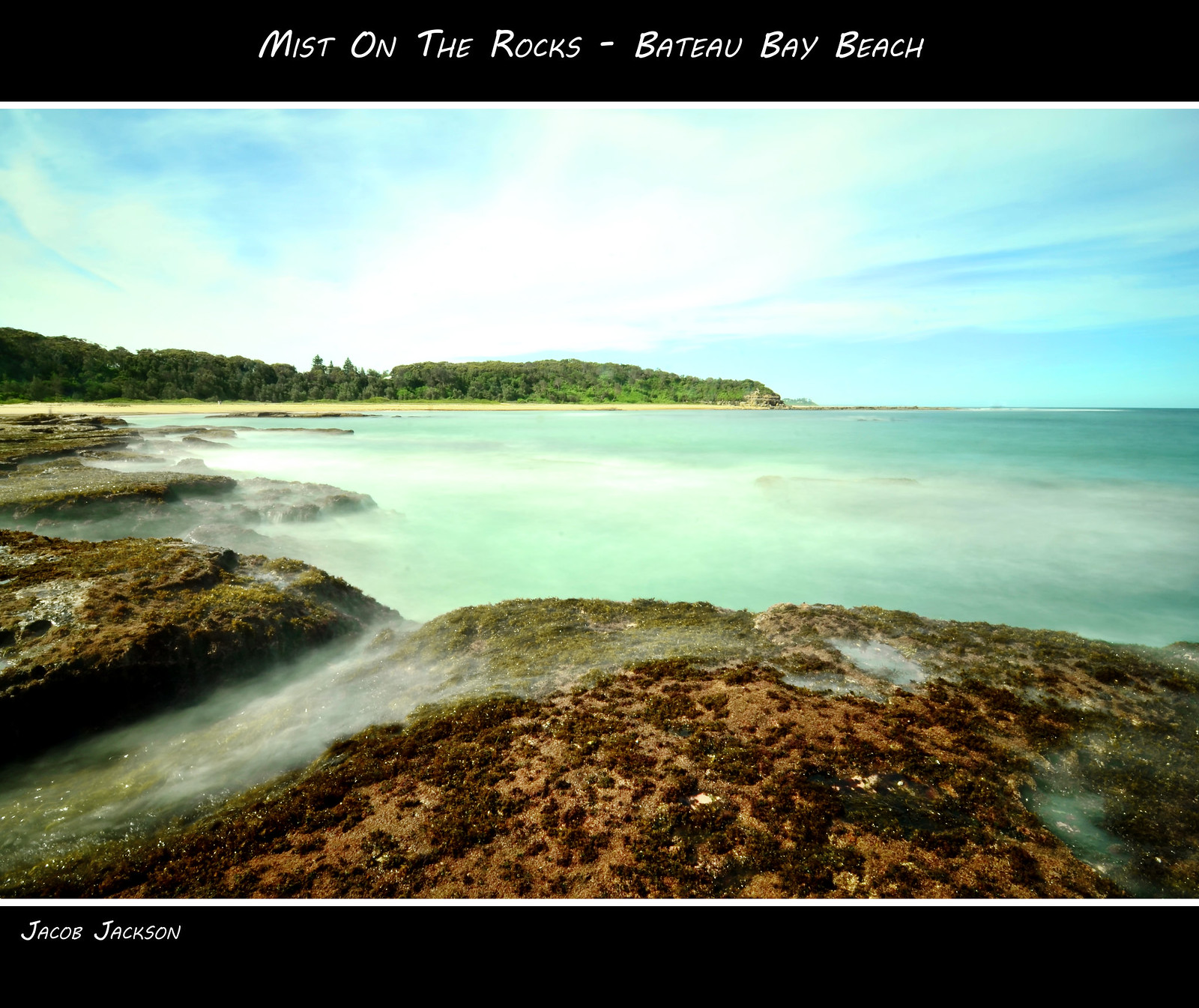A photograph captures a serene scene of Patau Bay Beach, framed by black borders at the top and bottom. The top border, with white text, reads "Missed on the Rocks, Patau Bay Beach," while the bottom left corner bears the name "Jacob Jackson." The image showcases a diverse coastal landscape. In the foreground, an area of dirt and rocks, layered with mist and dotted with seaweed, transitions into a sandy yellow beach stretching into the distance. To the right, a vast body of water shimmers in shades of green and blue. Overhead, a light blue sky is interspersed with thin, wispy white clouds. Beyond the sandy stretch lies a long line of green trees, rising almost like a hill, adding depth to the background.